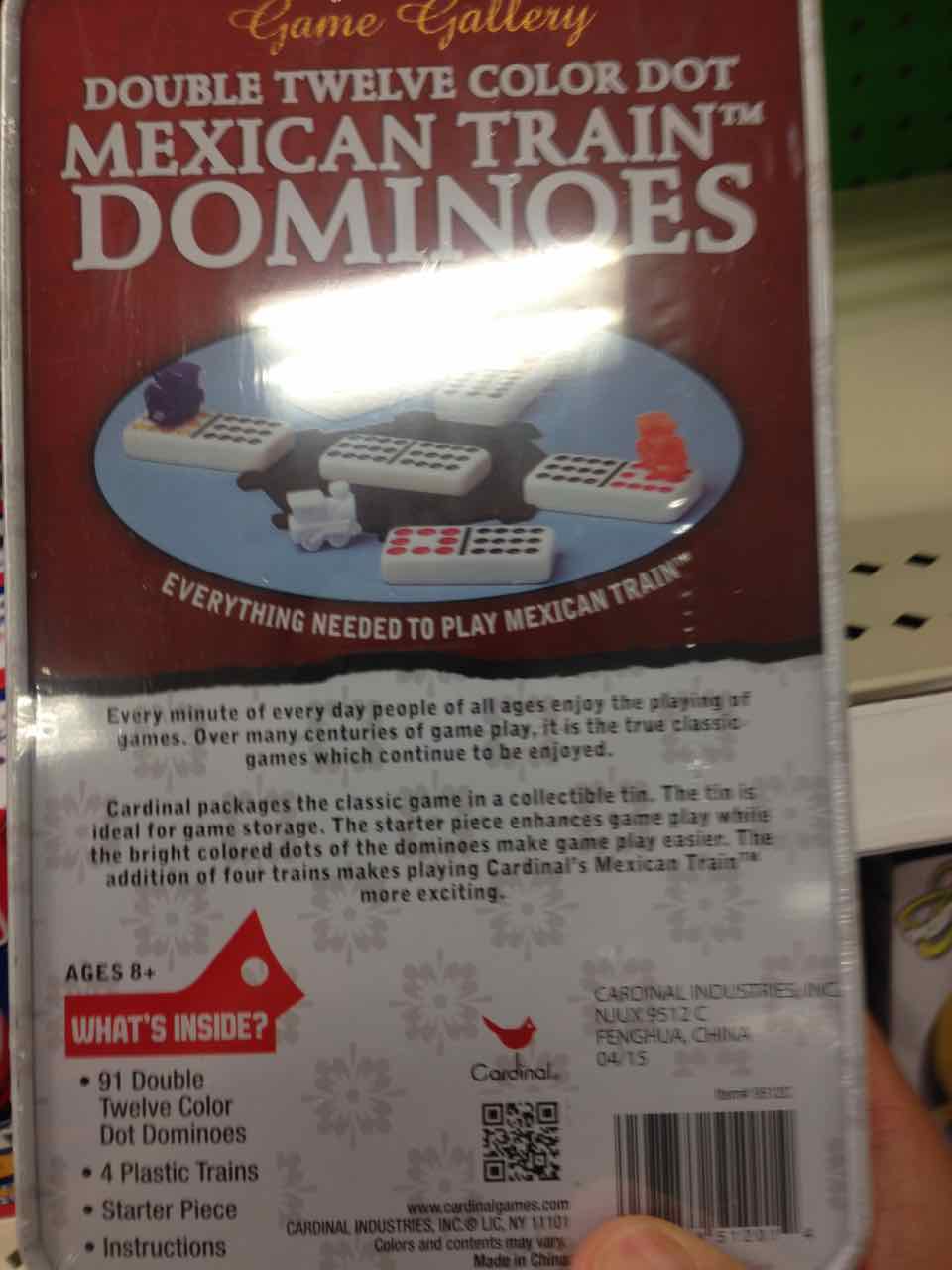The cover of the game package for Mexican Train Dominoes features a visually striking design with a red top half and a white bottom half, separated by a thin black strip. At the top, the name "Game Gallery" is prominently displayed in gold letters. Below that, in white letters, are the words "Double 12 Color Dots Mexican Train Dominoes." There is also a blue oval with a black ring encircling images of dominoes with various colored dots, a white train engine icon, and the phrase "Everything Needed to Play Mexican Train."

In the white section, there is a detailed write-up that reads: "Every minute of every day, people of all ages enjoy the playing of games. Over many centuries of gameplay, it is the true classic games which continue to be enjoyed." This is followed by "Cardinal Package is the classic game in a collectible tin. The tin is ideal for game storage," emphasizing the collectibility and practicality of the packaging.

To the left, a red area highlights the contents in white and black letters: "91 Double 12 Color Dominoes, Four Plastic Trains, a Starter Piece, and Instructions." Adjacent to this, the Cardinal Games logo, accompanied by a QR code and a partially visible barcode near the bottom right corner, rounds out the design. The cover also features a small thumb near the barcode, adding a touch of real-life interaction.